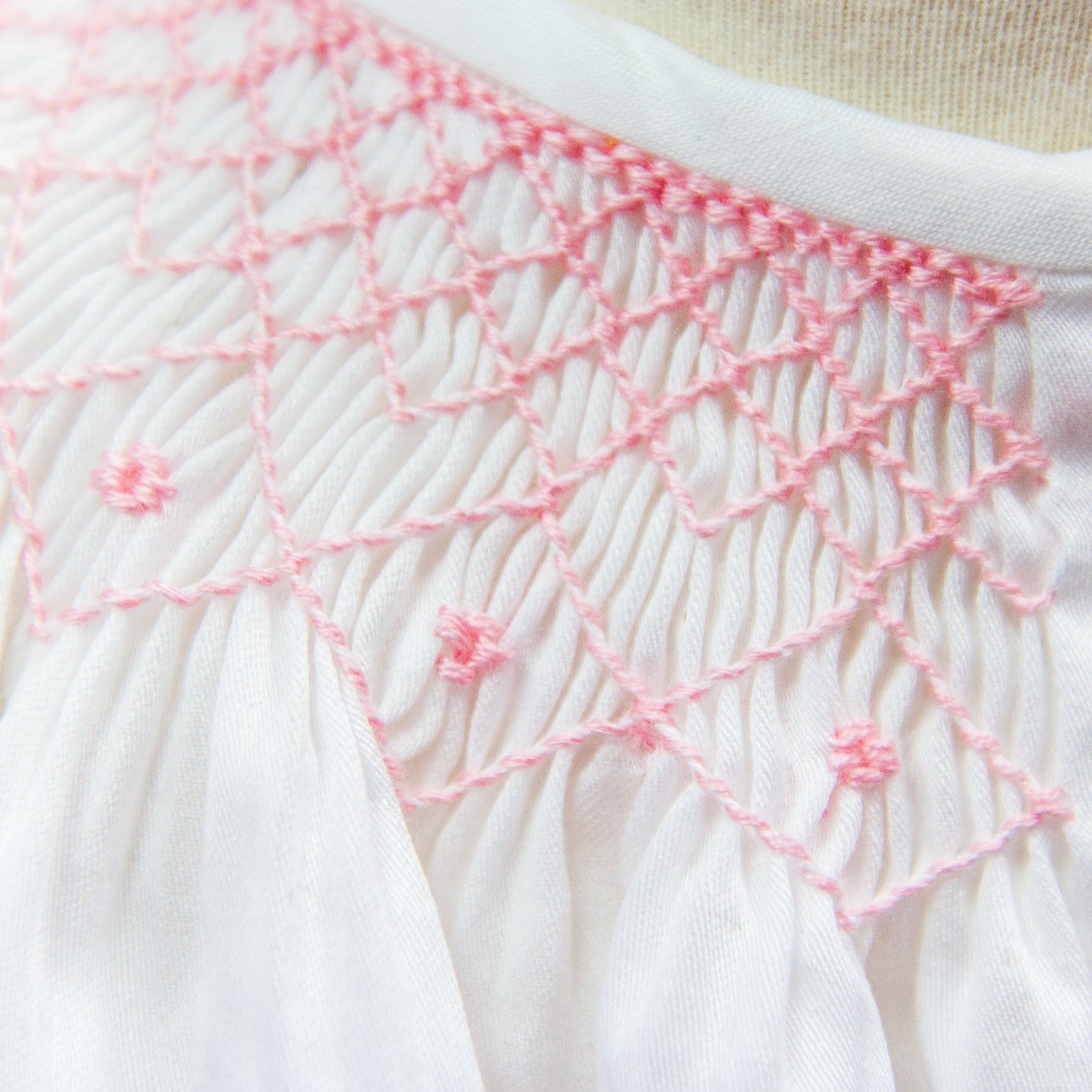This color photograph is a close-up of a detailed, knitted fabric that appears to be a garment, possibly a decorative dress, top, or baby clothes. The fabric is predominantly white and features a ruffled, stretchy knit texture, resembling a double knit material. The upper portion displays a delicate pink yarn intricately crocheted in a diamond lattice pattern, with the diamonds becoming slightly larger as they descend from the neckline. Each diamond's center near the lower middle of the image contains an embroidered pink flower. The top portion of the garment pleats near what could be the neckline, which curves off to the right of the image. There is a beige cloth backdrop visible at the top of the photograph. Emphasizing its ornamental nature, the absence of text, people, animals, and motorized vehicles suggests a focus purely on the intricate craftsmanship of the fabric.